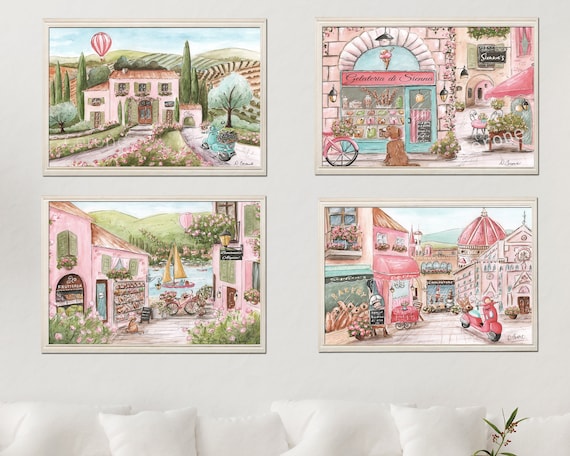This image features a white-walled living room decorated with four framed artworks arranged in a two-by-two grid above a white couch adorned with plenty of white throw pillows. In the lower right corner, the green foliage of a plant with small red berries peeks into view. Each piece of art is encased in a light cream or wooden frame and shares a cohesive cartoonish style with predominant shades of pink. 

The upper left painting depicts a whimsical manor house surrounded by trees and flowers, with orderly rolling hills in the distance and a distinctive red and white striped hot air balloon rising in the sky. The upper right artwork captures a lively street scene with pink awnings, a brown dog curiously looking into a storefront, an edge of a bicycle, and details like chairs from an outdoor cafe and an umbrella. 

In the bottom left, the scene features two pink buildings with a bicycle stationed between them, overlooking a serene body of water with a small sailboat and hills in the background. The bottom right image portrays another street scene, including a domed church, a bakery, a colorful scooter, and outdoor seating accompanied by a charming chalkboard sign depicting a chef’s face. Each artwork, evocative of Mediterranean village or town scenes, completes the cozy yet vibrant aesthetic of this living room.